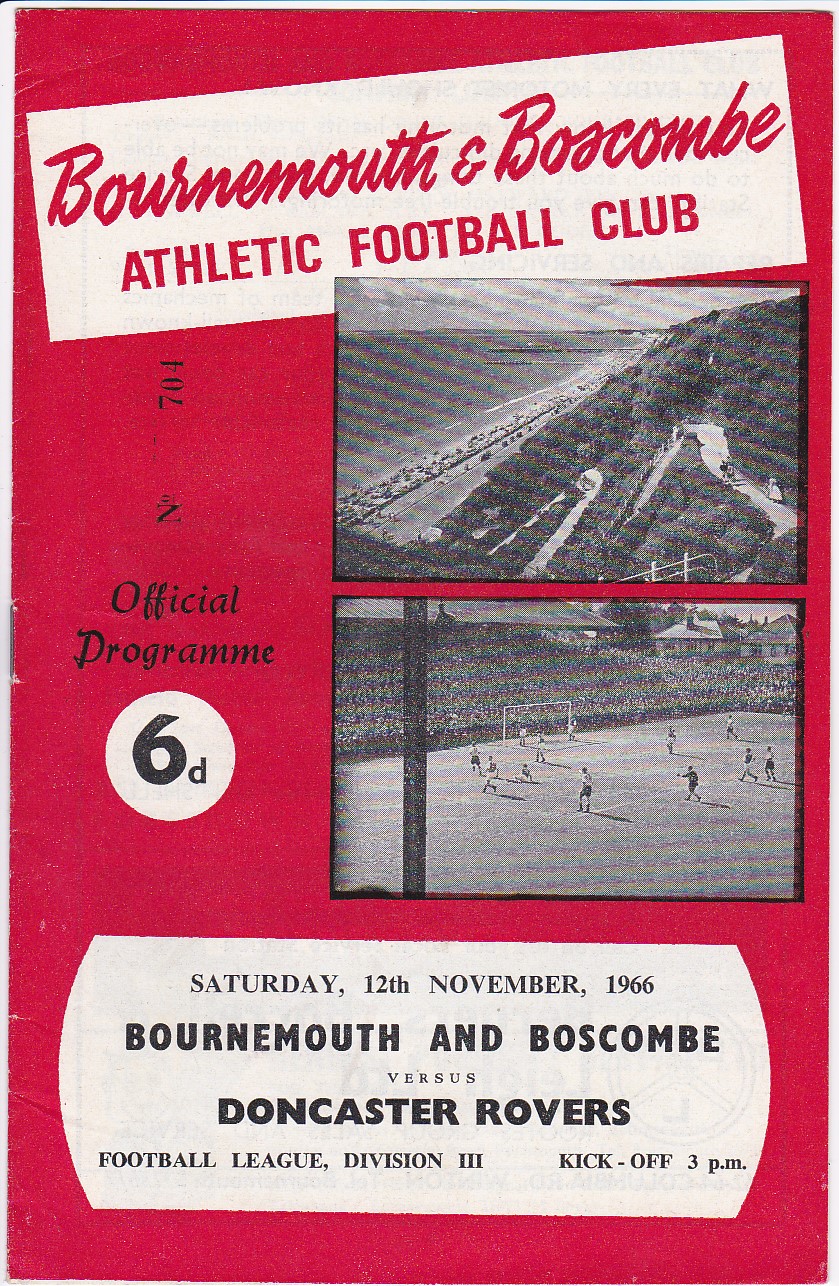The image is the cover of an old football (soccer) program from a British football club, primarily featuring a bold red background. At the top, in a white text box with red letters, it reads "Bournemouth and Boscombe Athletic Football Club." There are two black-and-white photographs: the top one depicts a scenic beach with mountains in the background, and the bottom one shows a football match with players on the field and spectators in the stands. To the left of these pictures, the cover text reads "Official Program 6d." Beneath this, in another section of text, it states, "Saturday 12th November 1966 Bournemouth and Boscombe vs. Doncaster Rovers Football League Division III kickoff 3 p.m."